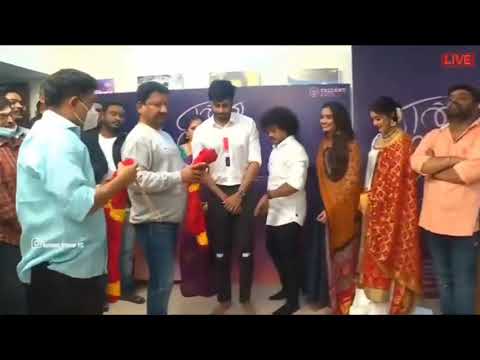The picture portrays a group of Indian people, likely captured during the COVID-19 pandemic, as visible by the presence of protective masks on some individuals. The scene is set in what appears to be an office environment, characterized by a purple and white wall adorned with posters and some advertising that is partially obscured by the people. In the upper right corner, the word "LIVE" is displayed in red text.

The main focus of the image is on two individuals at the front of the group, both holding a red and yellow fabric, possibly a jersey or a piece of traditional clothing, and facing towards the right of the picture. The man on the far left in the foreground is wearing a white elbow-length shirt, black pants, and a surgical mask, seemingly indicative of COVID-19 precautions. The other individual with him also appears to be examining or presenting the fabric.

Standing in line behind them, several people wear a mix of traditional Indian attire and casual clothing. For example, a man in blue pants and a tan shirt with crossed arms stands at the far right, looking somewhat disengaged, while another man with an untucked white button-down shirt and curly hair stands nearby. Among them, two women are dressed in flowing red and gold dresses, with one of them smiling and the other looking downwards.

The background also features additional masked individuals. One man has his mask pulled down beneath his nose, while another wears a blue mask partially lowered. The walls behind them, with their purple hue and white designs, run parallel to the line of people, creating a structured backdrop for the scene. Overall, the picture captures a moment of interaction or presentation, infused with cultural details and the reality of pandemic life.